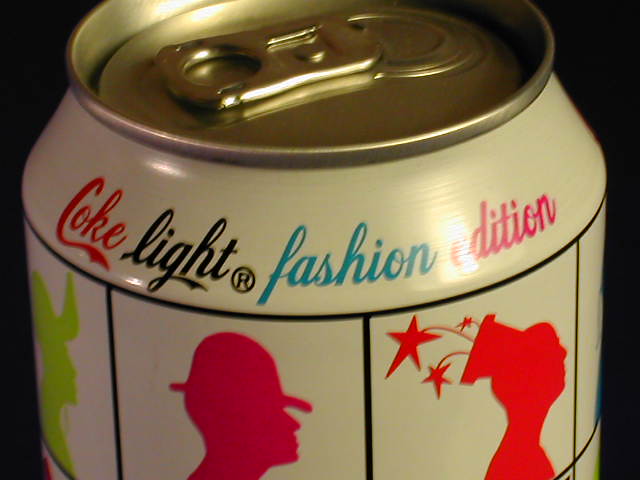The image showcases the top of an aluminum Coke Light Fashion Edition soda can. The can itself is off-white with the words "Coke Light Fashion Edition" prominently displayed near the top. The word "Coke" is written in red, "Light" in black, "Fashion" in light blue, and "Edition" in pink. The top features a standard silver pull tab. Below the text, three black-framed squares each contain a silhouette of a person's head. The left silhouette is a lime green figure resembling a cowboy, the center silhouette is a military man in dark pink, and the right silhouette, in red, features a person with stars emanating from their hat. This special edition can combines a retro aesthetic with unique, colorful profiles, making it a distinctive collectible item.